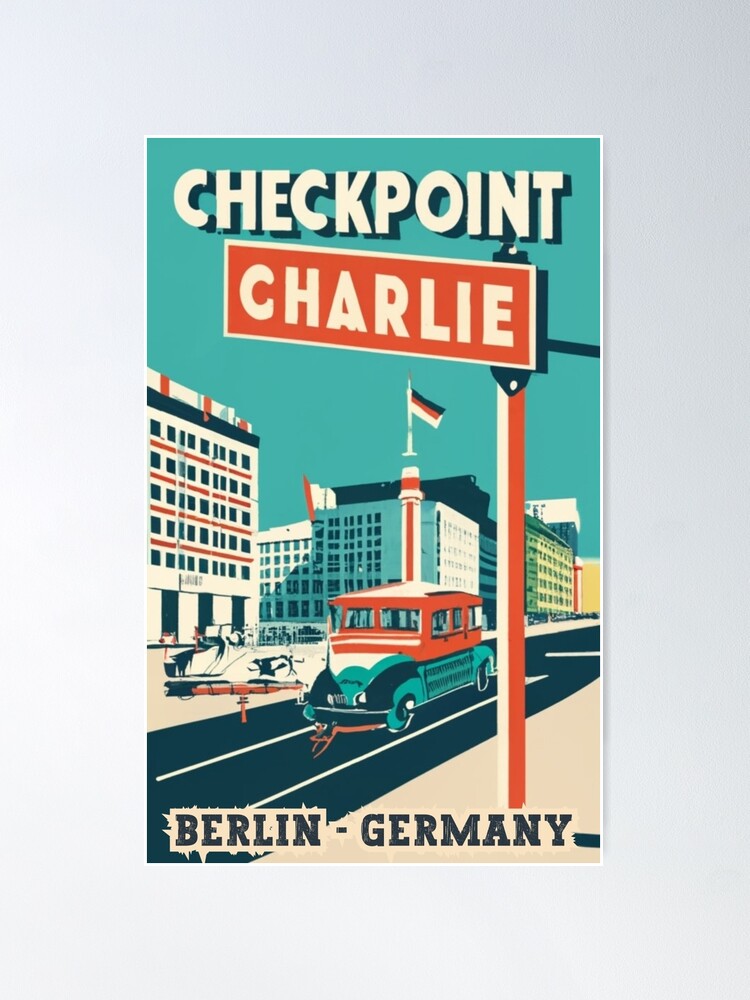This is a vibrant, Art Deco-style poster set against a teal background, framed with a thin white border. The top of the poster prominently features the words "Checkpoint Charlie," with "Checkpoint" in bold white font outlined in black, and "Charlie" in large white letters on a red rectangular background that resembles a street sign. Below, in black letters, it reads "Berlin, Germany." The scene depicted is a city street lined with tall buildings, some stark in shades of white, light blue, and gold, others with a touch of red or orange. A notable building at the top left corner displays a German flag. On the street, there is a vintage car with a distinct design featuring a light blue lower half and a red and white upper half, cruising along a black road with white lines. The cityscape in the background includes white buildings with numerous black-framed windows, and in some distance, a yellowish and gold-colored structure is visible. The entire scene brings a historical yet stylistic representation resembling the era around the 1940s.